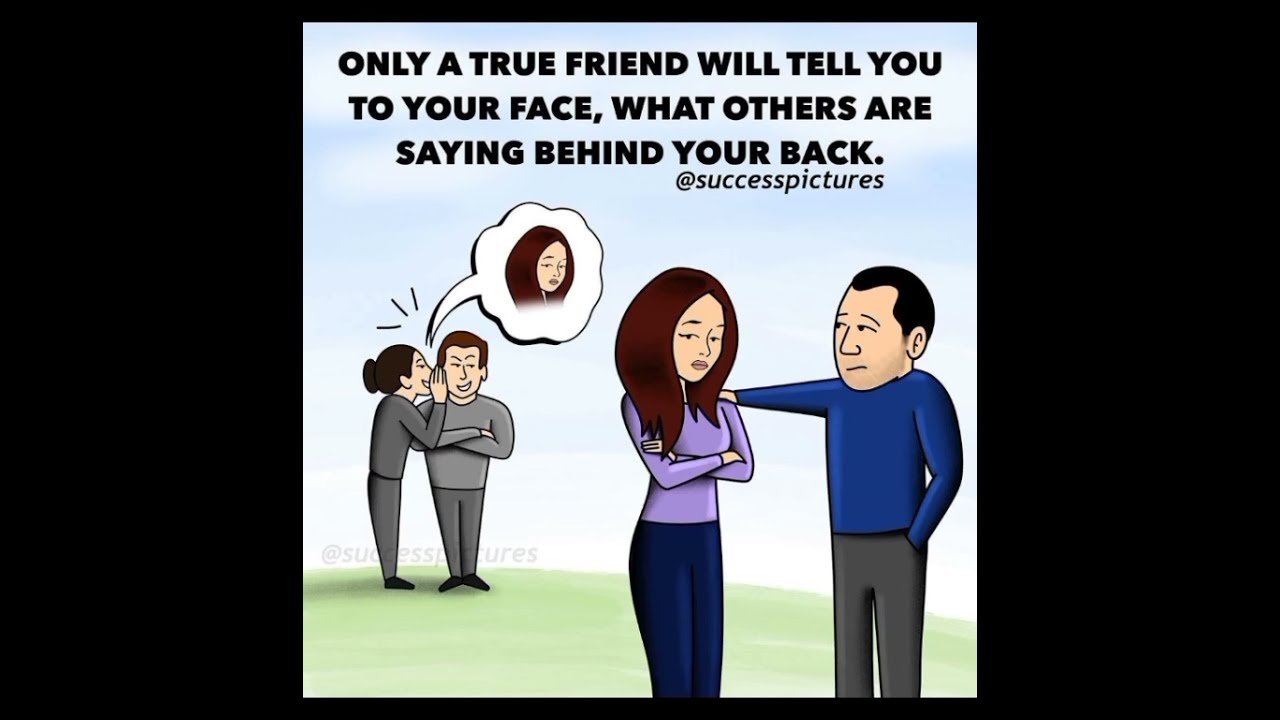The image is a cartoon set against a black background, designed to resemble a poster or announcement. In the center, against a light blue background, four people are drawn in detail. On the bottom right, a middle-aged man with short black hair, a blue sweater, and gray pants is facing left. He has his right arm outstretched, comforting a distressed woman beside him. She has long brown hair, is dressed in a purple shirt and blue pants, and is looking downward with crossed arms.

To their left, slightly in the background, stand two other figures. The man on the right has brown hair and is wearing gray with folded arms, while the woman on the left, dressed entirely in gray, has her hair tied up in a bun. She appears to be whispering into his ear, her hands raised to her mouth, with her face close to his ear. A speech bubble emanates from her whisper, depicting the exact face of the distressed woman in the foreground, illustrating gossip.

At the top of the image, written in bold black uppercase letters, is the text: "ONLY A TRUE FRIEND WILL TELL YOU TO YOUR FACE WHAT OTHERS ARE SAYING BEHIND YOUR BACK." Below this text, in smaller print, is an at sign followed by "SUCCESS PICTURES." This image serves as a caution against rumors and highlights the significance of true friendship.